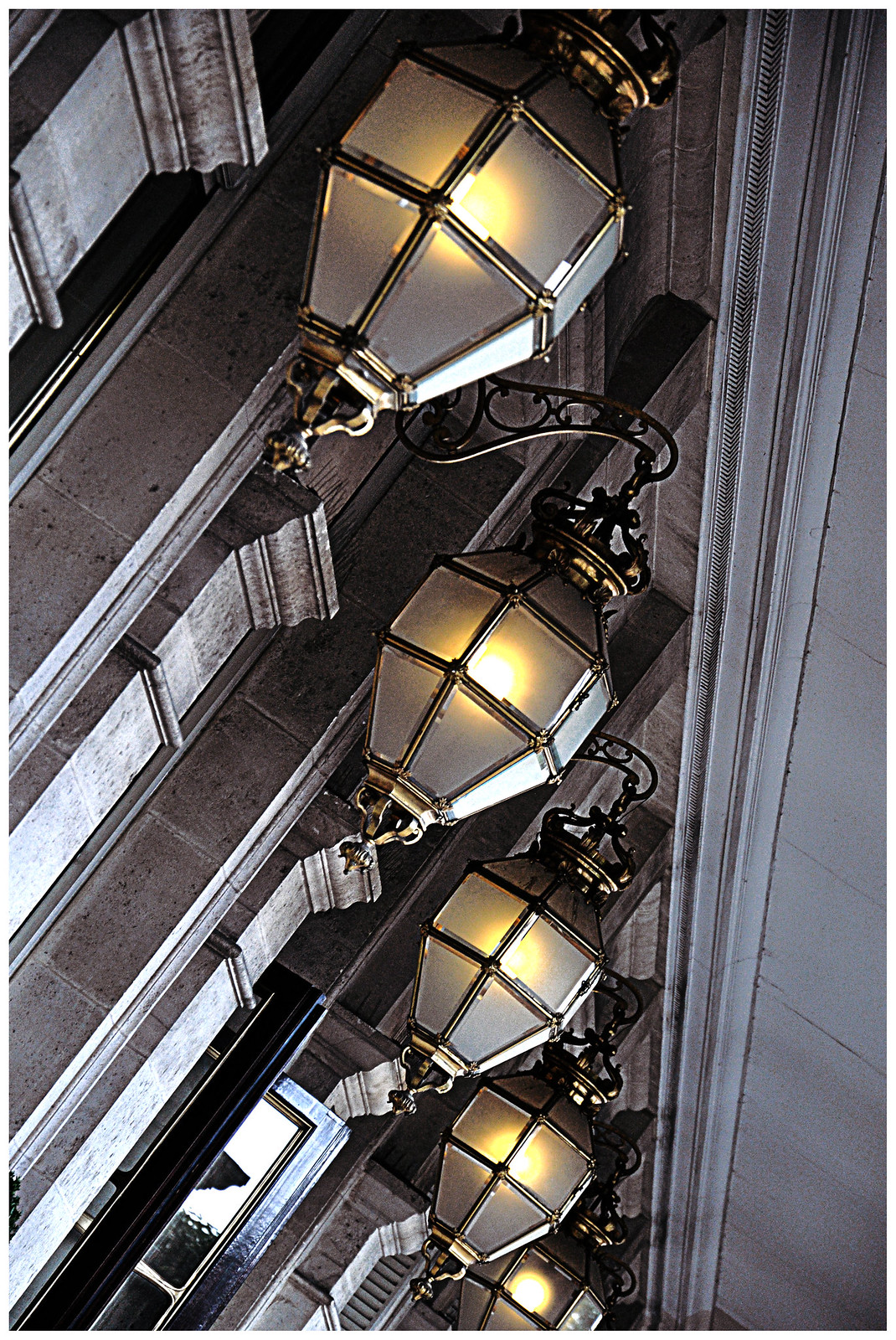This image captures an intricately designed row of five hanging lanterns, possibly adorning a well-architected building. The photograph, taken from a tilted angle looking upwards, presents these elaborate light fixtures in a vertical alignment down the center of the frame. Each lantern is a sophisticated blend of frosted glass panels—square in the middle, transitioning to a triangular shape at the bottom—meticulously edged in gold. The lanterns are suspended from ornate gold arms with curlicued designs, culminating in an elaborate, sculpted gold base. The background reveals large stone columns, likely white marble but aged and dirty, supporting the structure. The ceiling visible above is decorated with grey lines and patterns, matching the overall grey tone. Additionally, black doors with golden frames can be seen midway through the row of lanterns. The photograph does not include any text and features a color palette primarily of gray, gold, and white. The setting could be either indoors or outdoors, as the architectural elements blend seamlessly.